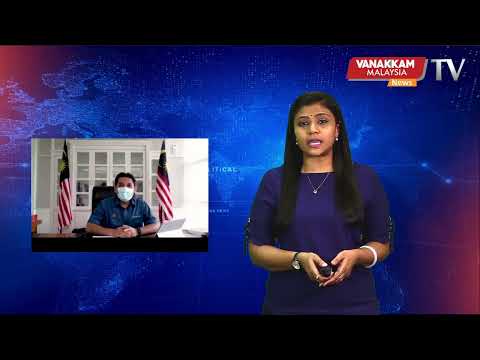The image features a television news broadcast titled "Vanakkam Malaysia," indicated by white text on a red rectangle and an adjacent "news" label in an orange box with white font, followed by "TV" in white text. The foreground showcases an Indian woman presenter wearing a long purple dress, adorned with a necklace, earrings, a watch on her right wrist, and a white bracelet on her left wrist. She holds a remote control with both hands in front of her. Her long black hair cascades down as she looks directly at the camera. The background is predominantly blue with hints of purple in the lower right and upper left corners, featuring an illustrated globe. To the left, there is a smaller inset picture, appearing like a live stream, of a man in a short-sleeve dark blue or denim shirt, seated at a black desk, wearing a white medical mask, with his hands folded. Behind him are two red and white striped flags with a blue section, against a backdrop of white windows. The man seems to be a government official, possibly being interviewed by or featured in the broadcast.